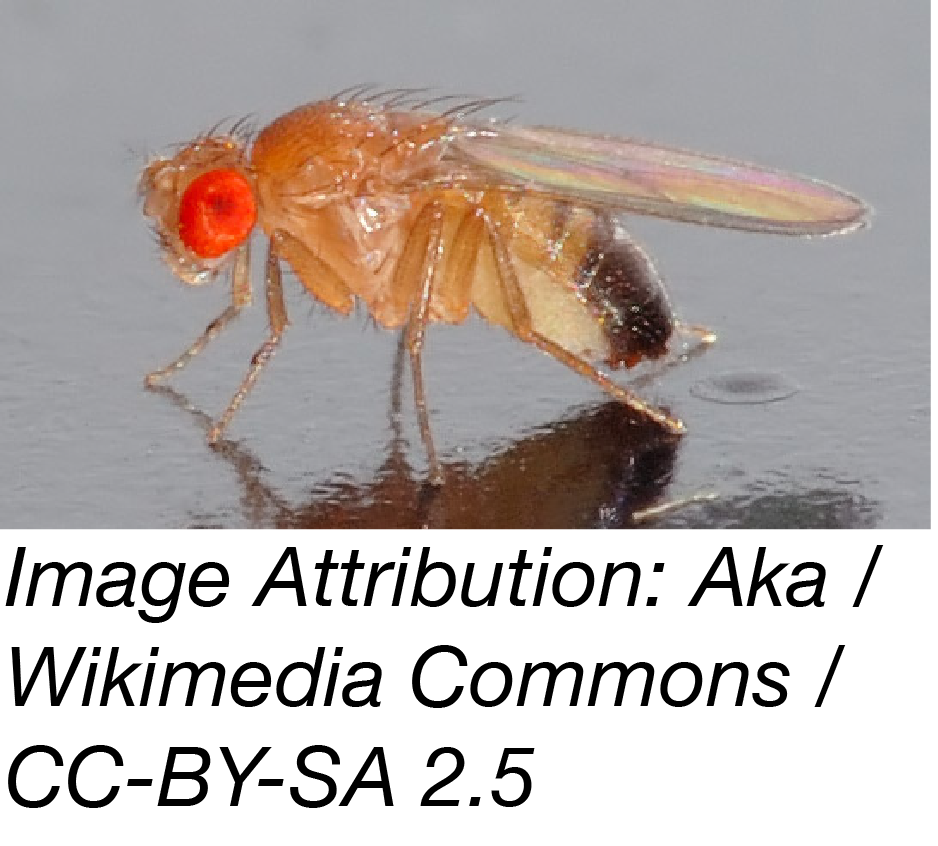This is an extreme close-up photograph of an insect, likely a fly, with specific details highlighting its appearance and the surrounding elements. The insect, depicted in tones of tangerine orange to orangish-yellow, is prominently featured in the center of the image. It has a strikingly large, bright red eye that is multifaceted, characteristic of flies. The insect's body is covered in small hairs protruding from its back and head, adding texture to its appearance.

It has a total of six visible legs, although the precise number is obscured. The creature's wings are thin, translucent, and display a subtle, rainbow-like sheen. One wing is especially visible on the left side. Its abdomen is notably large with a gradient of colors, transitioning from tan to black.

The insect appears to be stuck on a wet, grayish surface, possibly flypaper or damp cement, which adds a reflective quality to the background. The overall setting suggests that the creature is immobilized. Below the insect image, there is text in large black letters against a white background that reads:

"image attribution: aka / Wikimedia Commons / CC-BY-SA 2.5."